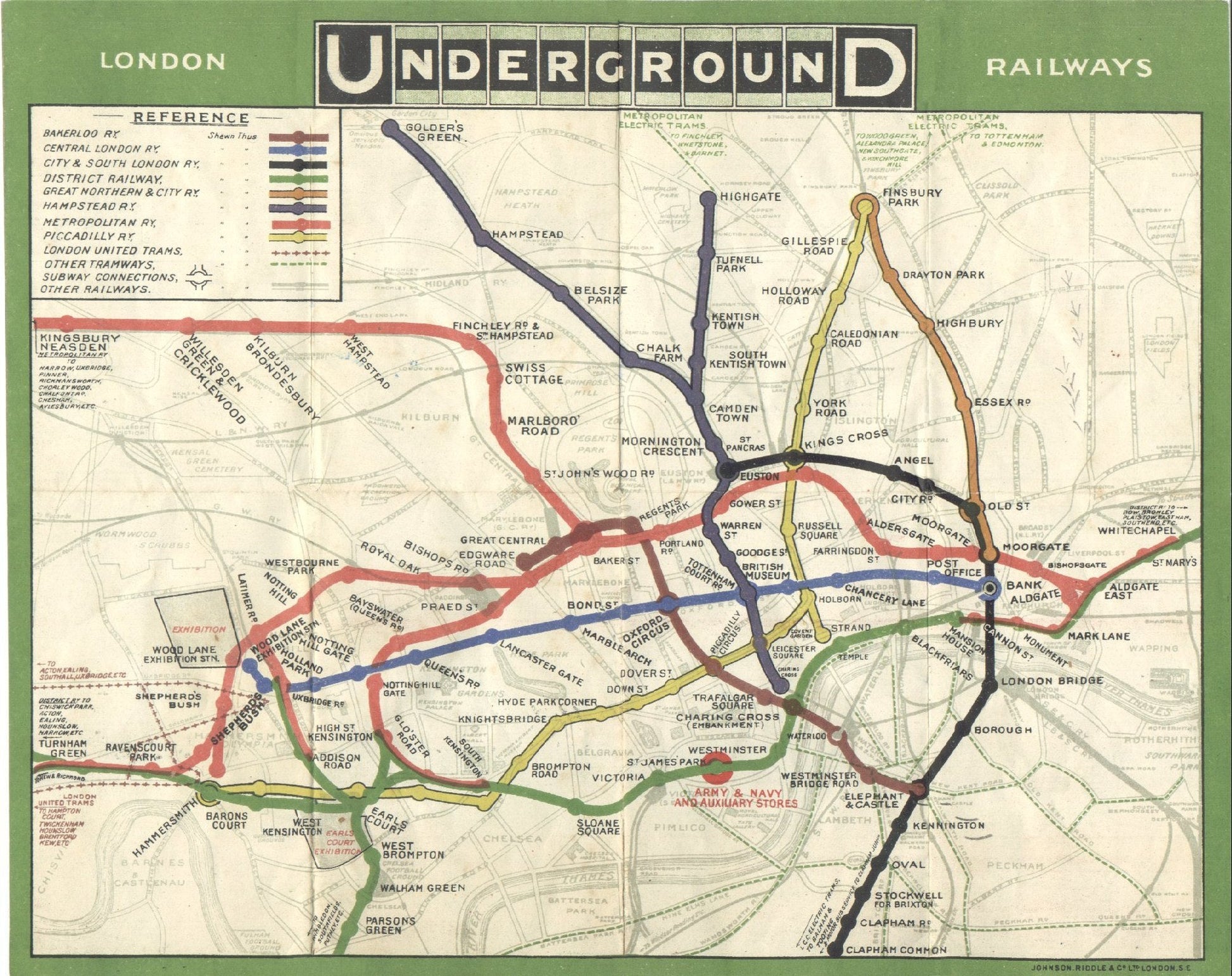This image is a detailed map of the London Underground Railways, designed as an older poster or advertisement. The top of the map prominently reads "London Underground Railways" in white text against a black background. It showcases the different road routes, each depicted in distinct colors: brown for Barclay Road, sky blue for Central London Road, black for City and South London, green for District Railway, orange for Great Northern and City Rail, purple for Hampstead, red for Peak Daly, and yellow for London United Transit. 

The map includes a reference section explaining the meaning of each colored line. Subway connections are indicated with symbols resembling roundabouts, and tramways are illustrated with dotted lines. Key locations highlighted on the map include Lancaster Gate, Queen's Park, Bond, Army and Navy and Auxiliary Stores, Bank Oddgates, Highbury, York Road, and King's Cross, with London's Bridge appearing in the bottom right corner. The entire map is bordered in green, adding to its visual clarity and aesthetic appeal. The individual stops and routes of the London Underground Railway are central to the image, providing a comprehensive guide for navigating the city's transit system.